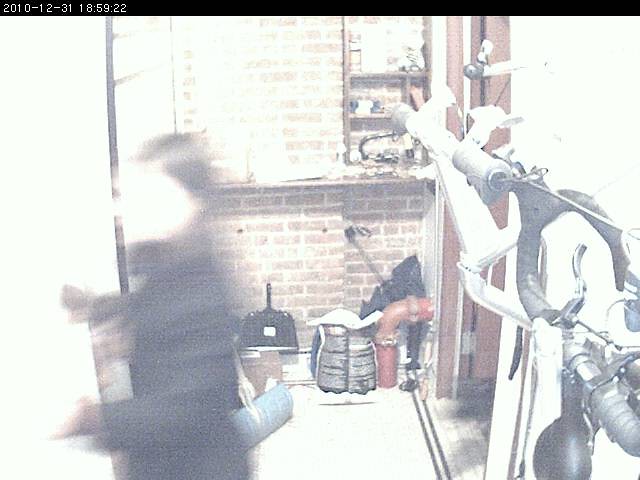The image appears to be a highly washed-out, grainy photograph likely taken with an older or security camera. A black banner across the top displays a timestamp in white text: "2010-12-31 18:59:22." On the left side stands a woman with long, tied-up black hair, wearing a black coat and carrying a blue purse over her shoulder. Her face is indistinguishable due to the blur and poor lighting, suggesting she might be in motion. The background features a brick wall with some shelving. On the floor, there's a collection of items, including a black dustpan, a black umbrella, and a black bag with white lines. Toward the right, there's a curved red pipe, potentially some plumbing, and what appears to be the handlebars of a bicycle. A doorway is visible to the left, and some objects hang from wires, contributing to the cluttered scene that might be a garage or a similarly purposed space.